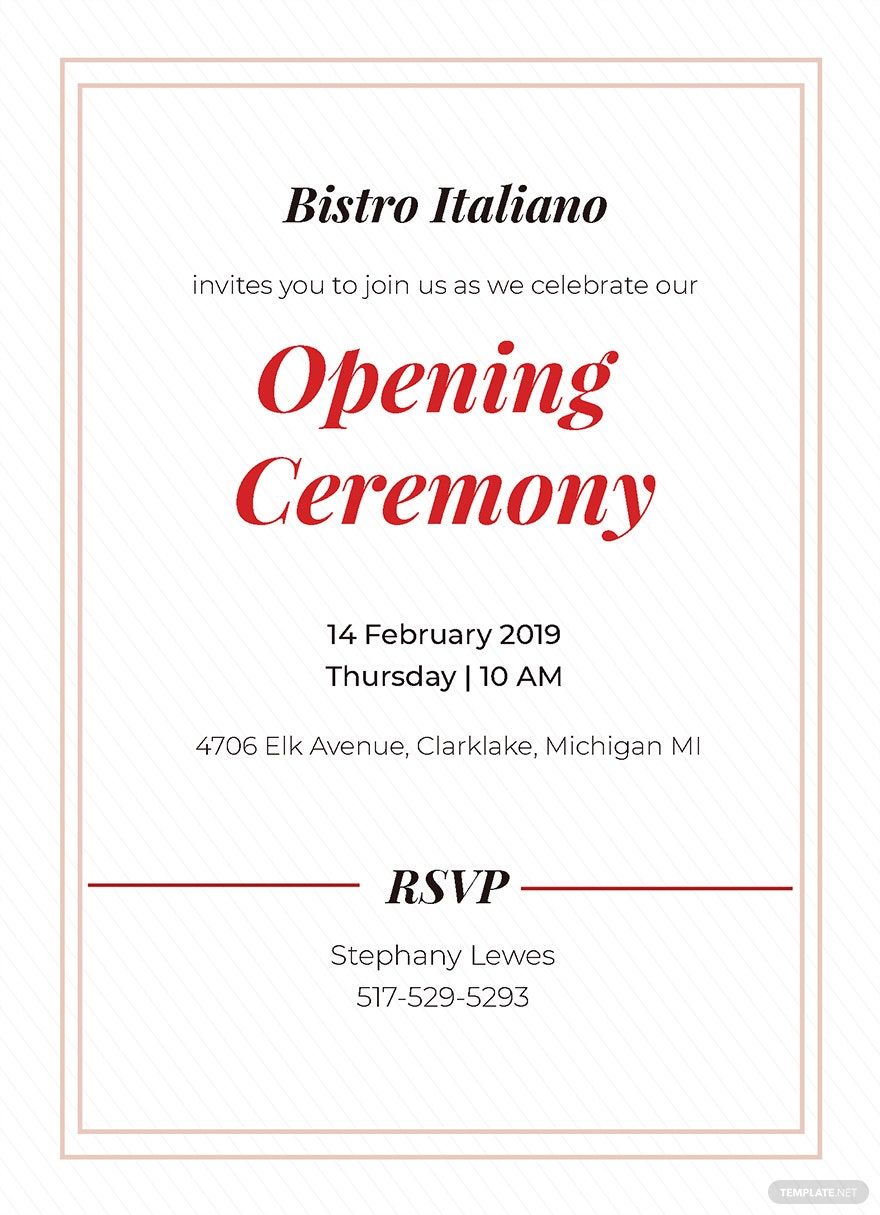This is an image of a formal invitation to the opening ceremony of Bistro Italiano, set in a clean, vertically-oriented card format. The card features decorative black text at the top, stating "Bistro Italiano," followed by the subtext, "invites you to join us as we celebrate our," leading into the larger, ornamental red text "opening ceremony." The date and time, "14 February 2019, Thursday, 10 a.m.," are clearly listed below in black. The address, "4706 Elk Avenue, Clark Lake, Michigan," follows. Toward the bottom, "RSVP" is written in bold black text, framed by red lines extending to the edges, with the contact details, "Stephanie Louise, 517-529-5293," below. The entire invitation is bordered by a double pink line, and the background features very faint lines that maintain readability.